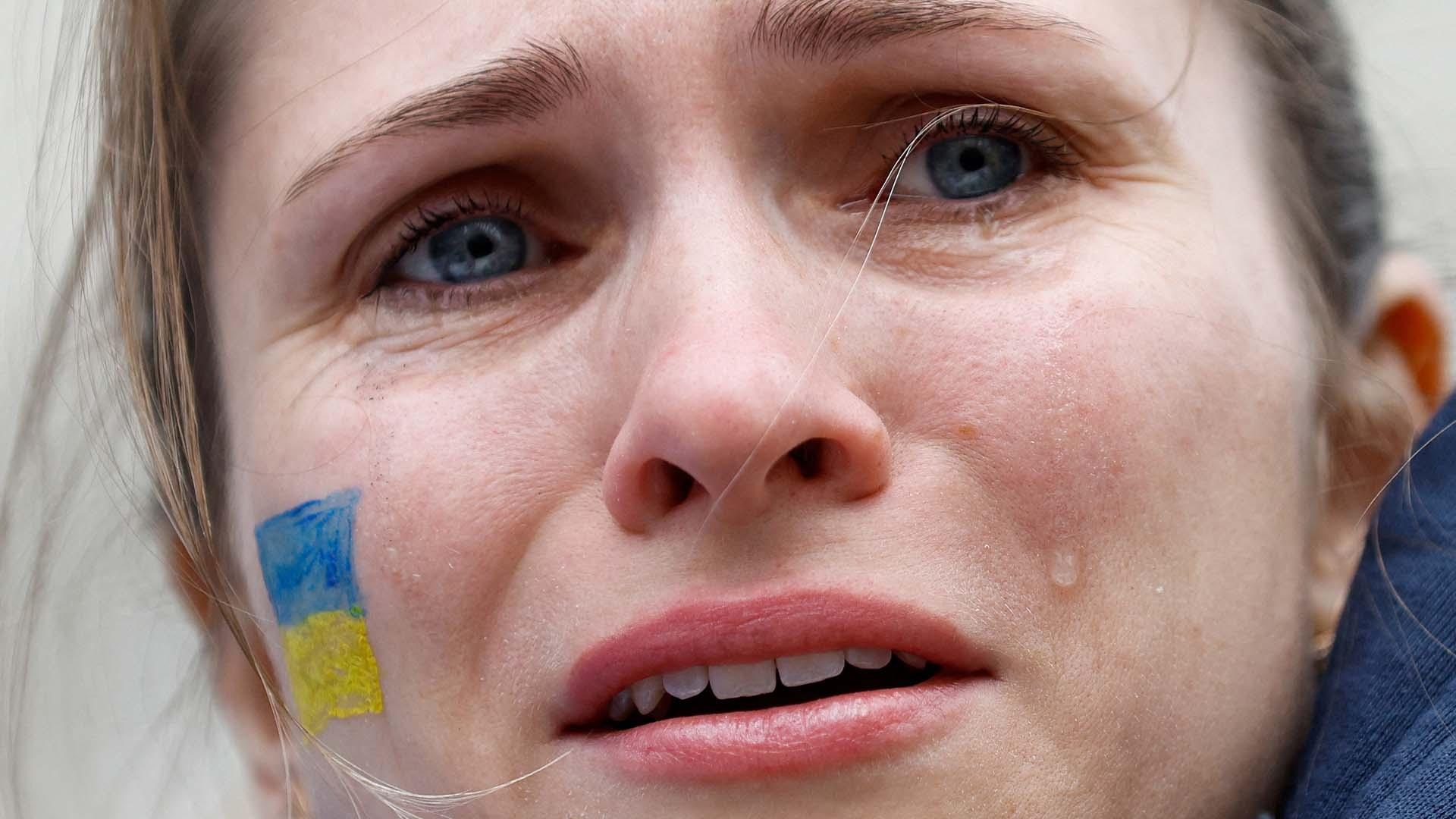This close-up photograph captures the anguished face of a middle-aged Caucasian woman, focusing on the area from her eyebrows to her chin. She possesses light blondish-brown, possibly short, hair and striking grayish-blue eyes. Her complexion is very light, and she wears a pinkish-peach lipstick. The expression on her face reveals deep distress: her eyebrows are furrowed, her mouth slightly open, and tears stream down her left cheek. On her right cheek, there is a two-inch painting of the Ukrainian flag, vividly displaying blue on top and yellow below, signaling her emotional involvement or support related to the Ukrainian-Russian War. The image encapsulates her sorrow and horror, potentially suggesting she is at a war protest or reacting to a traumatic event, with every detail emphasizing her profound sadness and concern.